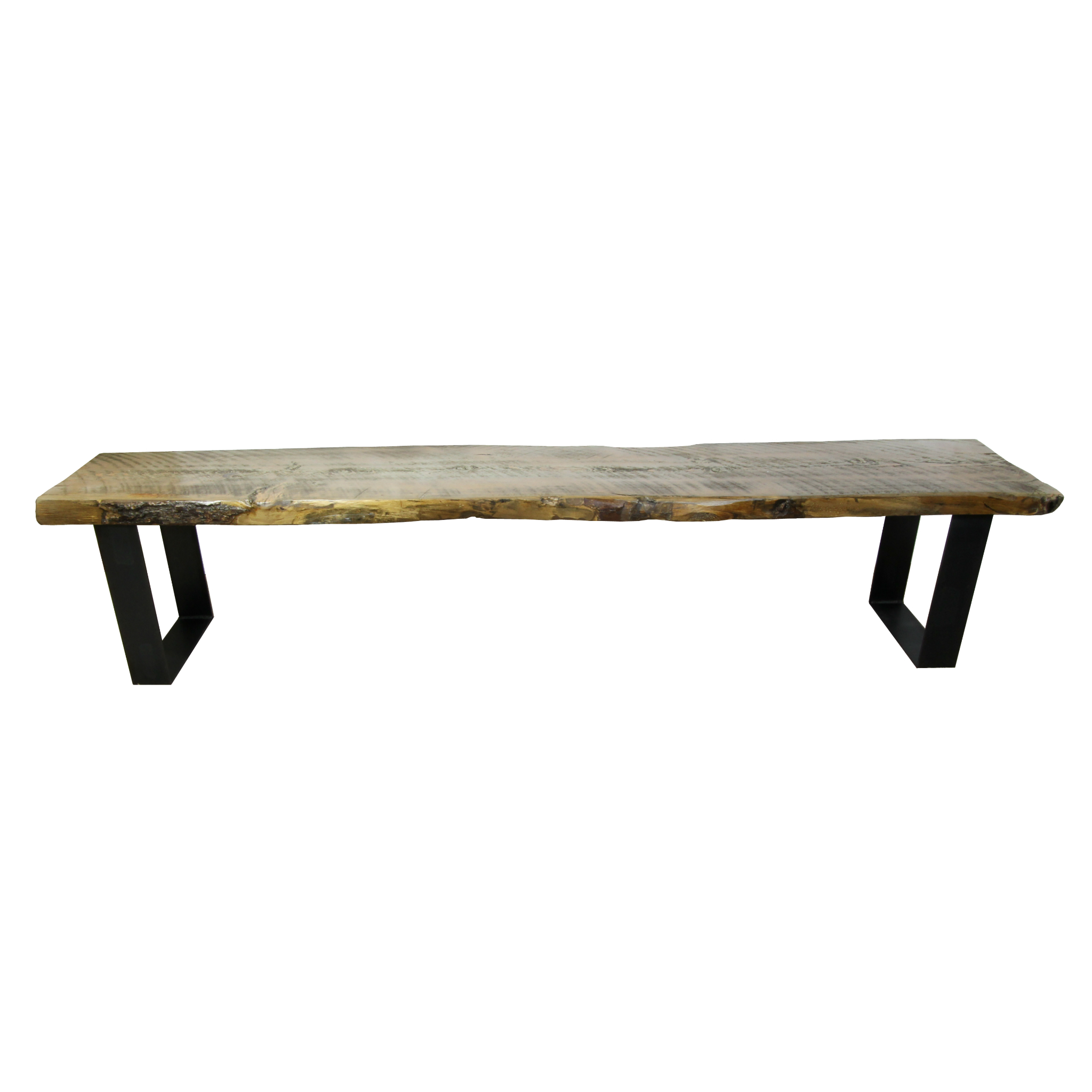The image features a simple wooden bench characterized by its raw, unfinished appearance, yet with a subtle gloss that adds a refined touch. Captured from an angle where the front side of the bench faces the camera, the photograph reveals both the top surface and the long, side profile. The bench's legs, one positioned at each end, are designed as hollow, square structures resembling the letter 'U' when viewed from the side. These legs are also wooden and bear a brown hue, harmonizing with the bench's natural aesthetic.